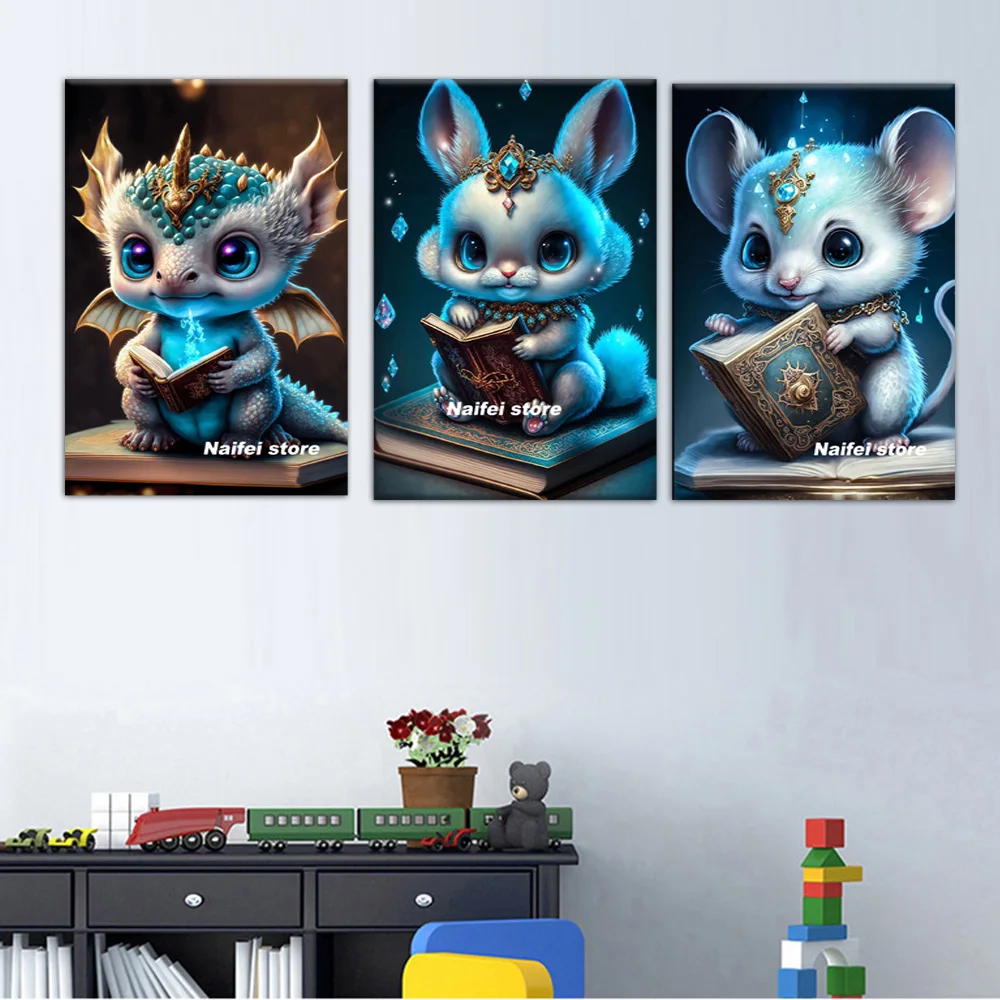This image portrays a colorful and imaginative child's room. In the bottom left corner, there's a black shelf adorned with a green toy train, a toy teddy bear, and a brown pot containing a fake flower. The shelf itself features black drawers with silver knobs. Centrally located within the room are two small children's seats—one blue and one yellow. To the right side, a vibrant tower built from child's blocks stands, showcasing a mix of red, green, yellow, white, and blue colors.

Above these playful elements, three whimsical themed renderings are displayed on the wall, each featuring a different animal character engrossed in a book. On the left, a baby dragon sits on a book with a flame emerging from another open book it holds. In the middle, a crowned baby rabbit is also seated on a book, holding another open book without any flame. The rightmost picture depicts a small bejeweled mouse reading a book while sitting on another. All three artworks contain white text that reads "Nefe store." The fantastical theme of these illustrations suggests they might be part of a children's story or television program.